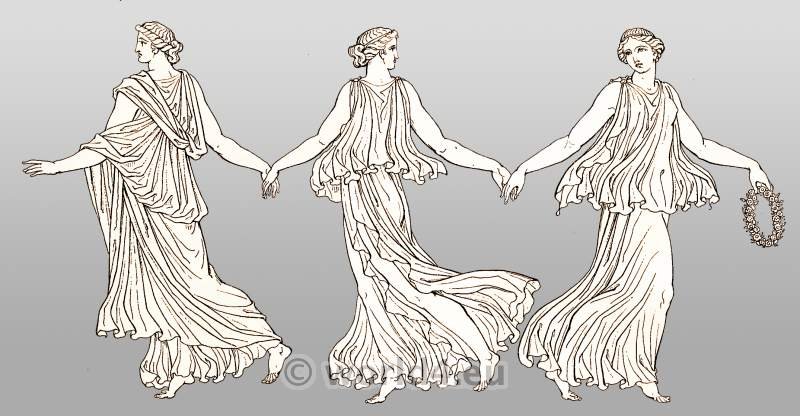The image depicts a detailed drawing of three Greek or Roman female figures, possibly representing the three Fates from ancient mythology. They are dressed in flowing, seamless gowns that reach their ankles, and their bare feet are visible. The figures are holding hands, with one figure positioned on the left, another on the right, and the central figure being gently pulled by the others. The central figure is turning away from the viewer but can be seen in profile, while the figure on the right, who is facing forward, holds a floral wreath. All three women have their hair braided and pinned up, adorned with headbands, and their classical features suggest they are idealized forms of ancient goddesses or mythological characters. The background is a muted gray, accentuating the marble-white appearance of the figures, and the clothing and hairstyles are reminiscent of traditional Greek or Roman attire. The bottom of the image features a watermark with "copyright world war dot mu," and the drawing, executed in an ink or pencil style, gives the scene a fluid, dynamic motion as if the figures are dancing. The entire composition measures approximately twelve and a half inches wide by seven inches tall.